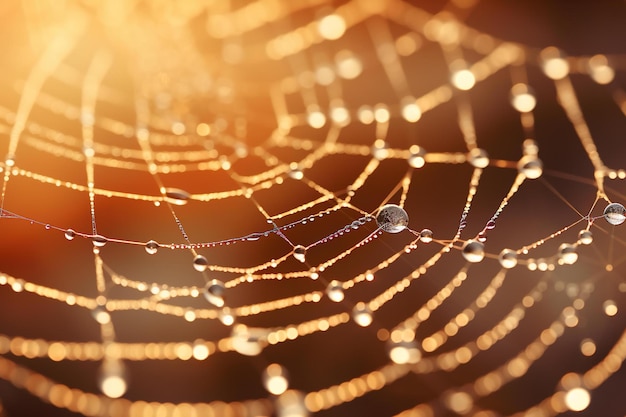This is a color photograph showcasing a close-up view of a spider's web adorned with glistening morning dew drops. The photographer has masterfully captured the intricate details, with each water droplet clearly visible. The web is partially in focus, especially near the bottom where there is a particularly large dew drop that stands out due to its size and the glow from the sunlight. The sunlight, emanating from the top left of the image, casts a beautiful, golden hue that illuminates several of the water droplets. The web itself curves and spreads wider towards the right, with droplets varying in size from large to very tiny, creating an intricate, sparkling pattern. The background features a muted brown color, providing a subtle contrast that highlights the delicate beauty of the spider's web.